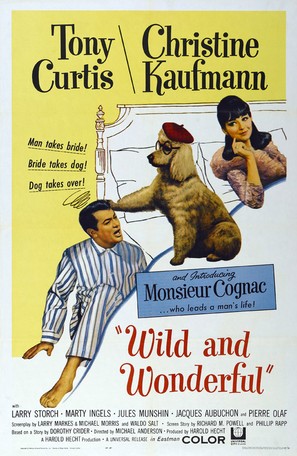This vintage movie poster from the 1940s or 1950s, titled "Wild and Wonderful," features Tony Curtis and Christine Kaufman. At the top, the names "Tony Curtis - Christine Kaufman" are prominently displayed. The centerpiece illustration depicts a whimsical scene: a woman, in color, is lounging on a black-and-white drawn bed, her hand gracefully touching her cheek as she gazes to her right. By her side, a dog sits comfortably on the bed, adorned with glasses and a red artist's cap. The dog appears to have pushed a pajama-clad man off the bed, who is now seated on the floor beside them. Surrounding the scene are humorous taglines like "Man takes bride, bride takes dog, dog takes over." Below, in blue lettering, it reads "Mansoor Konak who leads a man’s life," followed by "Wild and Wonderful" in quotes. The background towards the top is colored in a goldish-yellow hue, adding to the nostalgic feel of the poster. At the bottom, it displays the cast in smaller font, further highlighting the whimsical dominance of the dog in this comedic film.